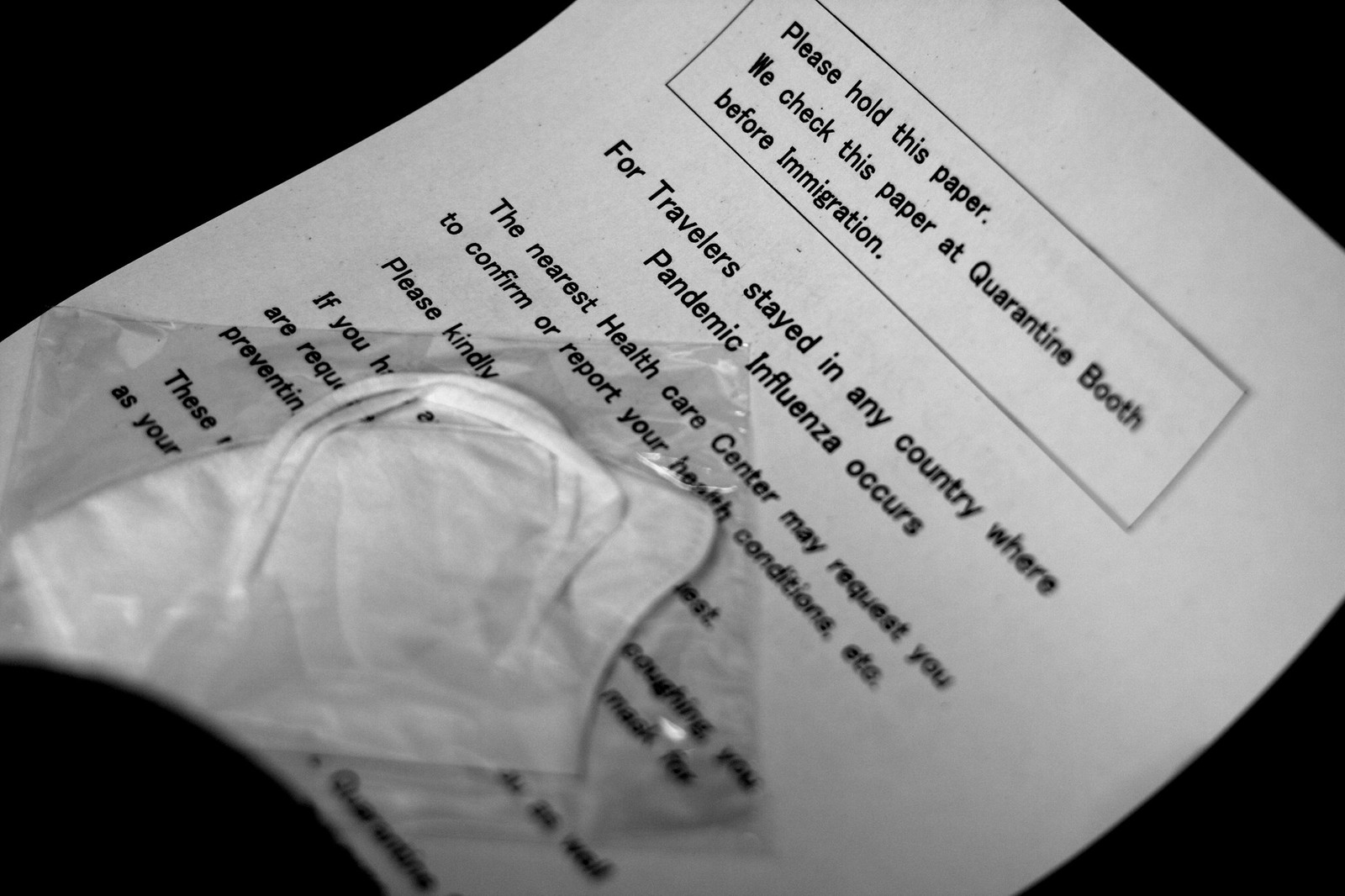This black and white image features a piece of paper against a black background, partially covered by a white face mask enclosed in a cheap, clear plastic bag. The paper contains critical information, primarily legible in the top section. The text reads: "Please hold this paper. We check this paper at the quarantine booth before immigration. For travelers stayed in any country where pandemic influenza occurs, the nearest healthcare center may request you to confirm or report your health conditions." Further text is obscured by the face mask, making it indecipherable. The paper appears slightly elevated at an angle, either due to the contours of the mask or the angle from which the photograph was taken.